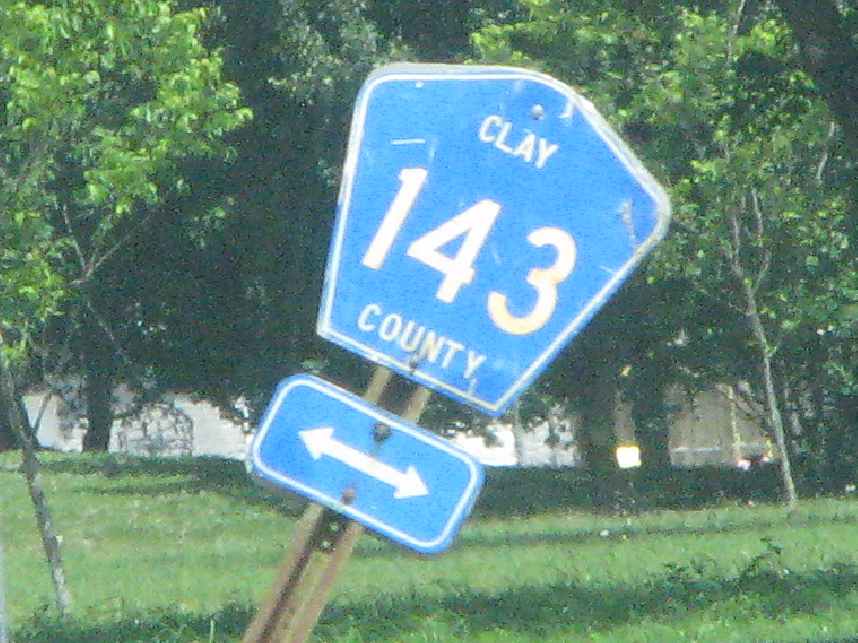A daytime photo captures a blue roadside sign reading "Clay 143 County" with a double-sided arrow pointing left and right. The signpost leans slightly to the right. The background features a grassy area followed by a line of trees, enhancing the natural setting of the scene.